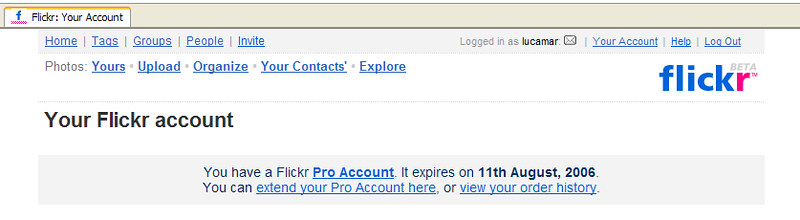The image is a detailed screenshot of the Flickr account page, displaying a webpage with a white background and a gray bar at the top. In the top gray bar, there is the Flickr logo, with the letter "F" in blue followed by "L-I-C-K-R," and the "R" is in pink. The bar reads "Flickr: Your Account" and belongs to a user logged in as 'Luke Kumar.'

Below the top bar, there are several blue, underlined navigation links: "Home," "Tags," "Groups," "People," "Invite," "Your Account," "Help," and "Log Out." Adjacent to these links is an email icon represented by a small envelope.

A second row of similar blue, underlined links includes options for: "Photos," "Yours," "Upload," "Organize," "Your Contacts," and "Explore." On the right side is the Flickr logo again, with the same color scheme as mentioned previously, followed by the text "Your Flickr Account" in black.

Towards the bottom of the page, there is a gray highlighted section stating: "You have a Flickr Pro account. It expires on 11th August 2006." It offers options to "extend your Pro account here" or "view your order history," both links being in blue.